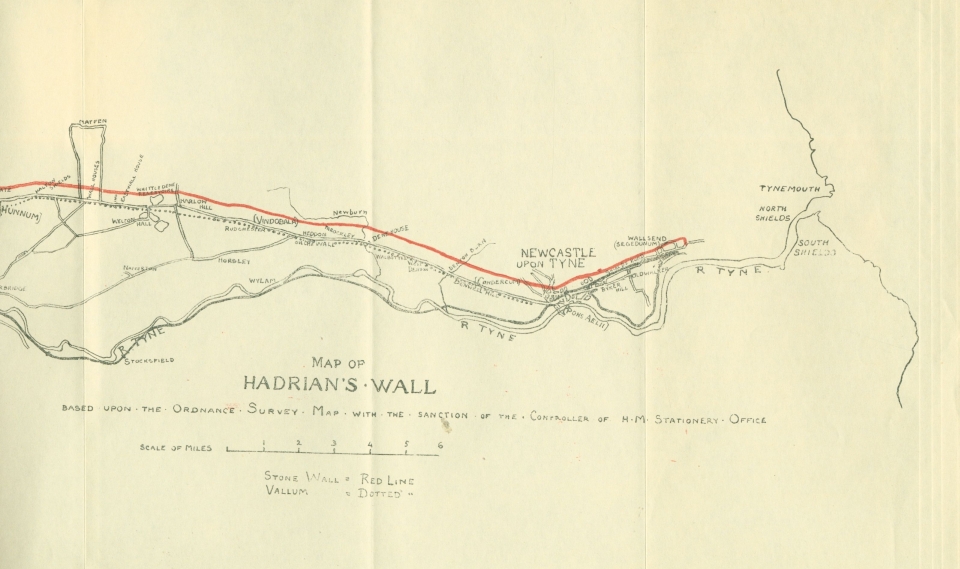The image features a vintage, worn, and repeatedly folded map drawn in pencil and black ink on a cream or off-white piece of paper. This map, identified as a "Map of Hadrian's Wall," is based on the Ordnance Survey map and includes the sanction of the Controller of the HM Stationary Office. The main elements of the map are depicted with black lines, while a prominent red line, indicating the stone wall, traverses it. Notable geographical and topographical features such as the River Tyne and Newcastle upon Tyne are clearly marked. The bottom of the map provides a key, including a scale of miles ranging from one to six, which explains the red and dotted lines representing the stone wall and volume, respectively. Despite some of the text being ineligible, the map details numerous trails, a coastline, and mountainous regions, delivering a comprehensive depiction of the landscape surrounding Hadrian's Wall in England.